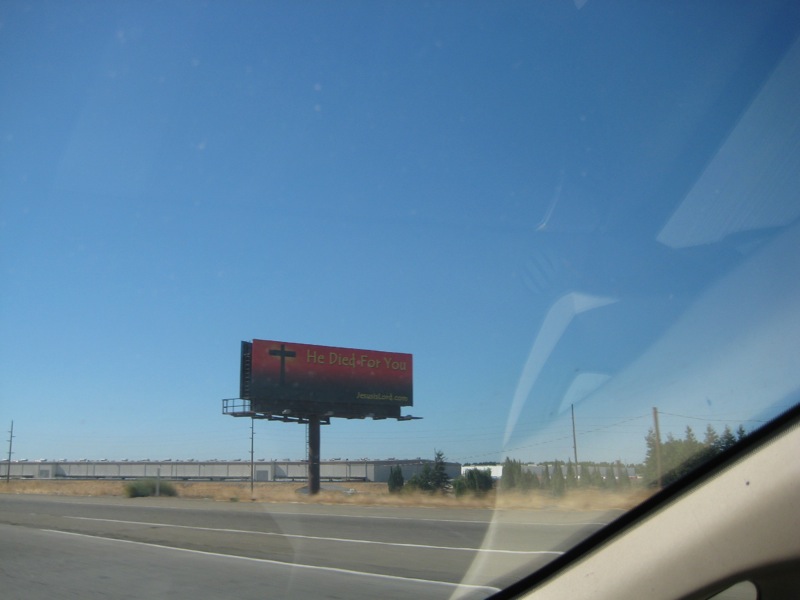This color photograph, captured from inside a moving vehicle on a highway, showcases a bright, cloudless blue sky. The scene is lit by daylight, and the bottom portion of the image includes the car's windshield, which reflects part of the tan interior. Positioned slightly to the left of the center is a large roadside billboard. This red billboard, which fades to black in the middle, bears a prominent yellow text that reads, "He died for you." To the left of this text is a silhouette of a cross, suggesting a religious message, possibly related to a church. The smaller text in the bottom right corner of the billboard is blurred and unreadable. In the background, a single-story, factory-like warehouse stretches to the back left of the image, reinforcing the industrial feel of the scenery. The surroundings include green trees and dried brown grass, contributing to the sense of a broad, open landscape typical of North America. White lines mark the gray highway, indicating the vehicle is in motion.